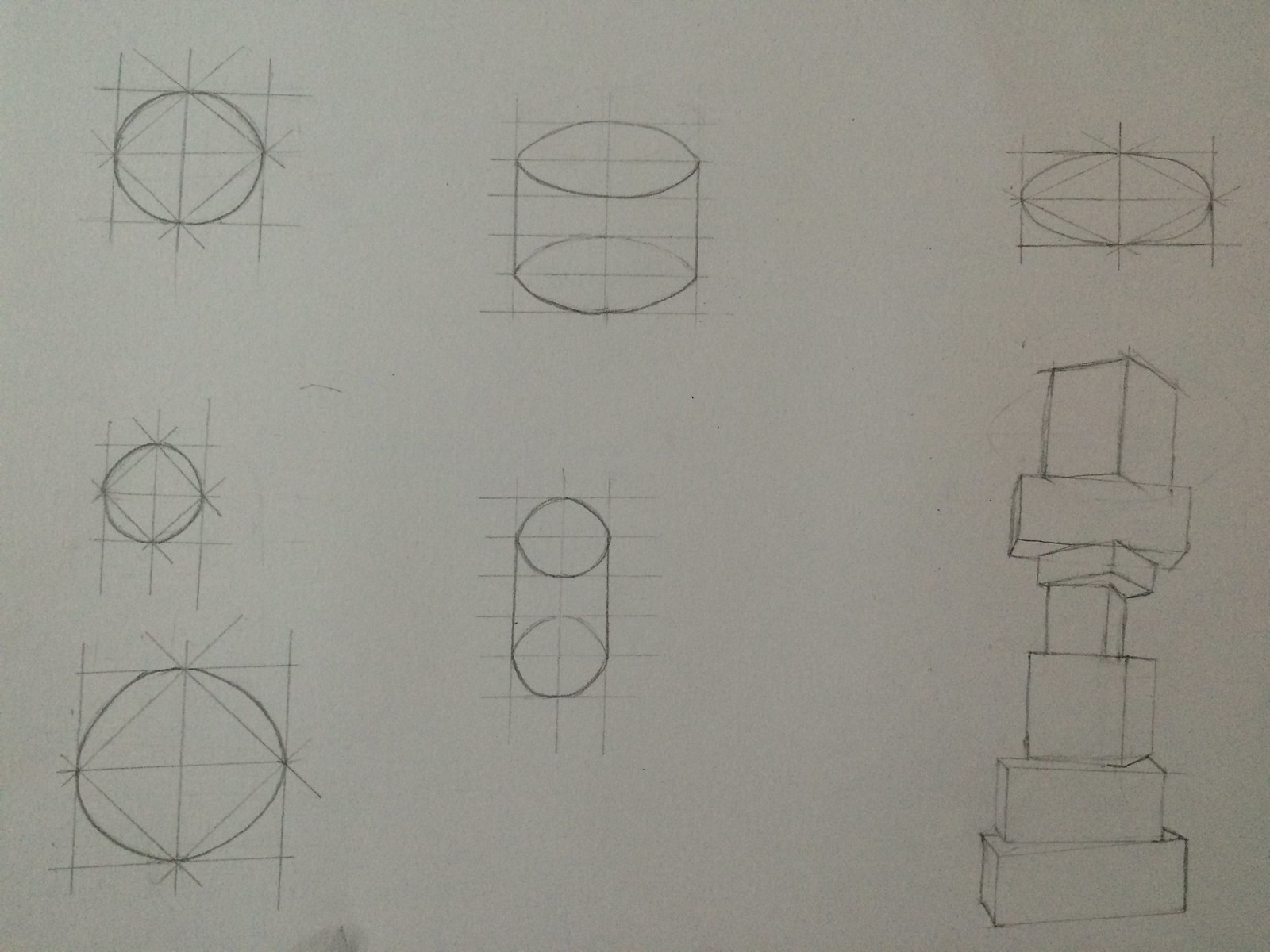This image showcases a detailed sketch of seven different geometric designs. The first design is a circle with multiple intersecting lines running across, through, and around it. Inside this circle, there is a smaller square and a plus sign. Below this, the second design mirrors the first with a circle and a tic-tac-toe pattern of lines intersecting it. The third design is a larger circle featuring a similar pattern, with lines intersecting in a grid-like manner forming squares within the circle. Central to the image is a cylindrical shape depicted in a 3D-like fashion, giving a sense of depth and a view around its entirety.